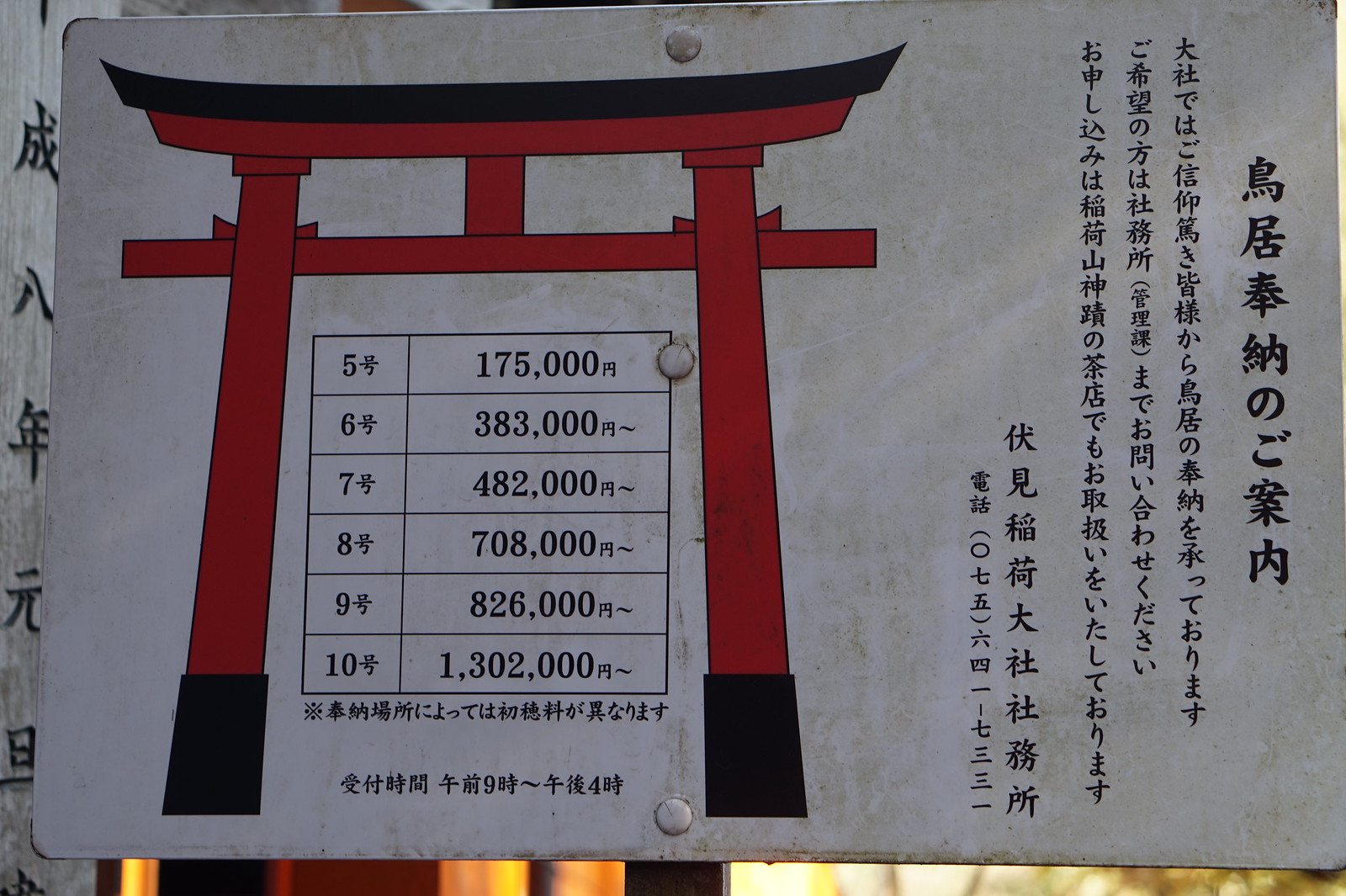This image is a close-up photograph of a rectangular white sign, which appears to be stained with brown marks. Prominently featured on the sign is a red and black illustration of a traditional Asian temple gate, or archway, consisting of two vertical poles connected by a horizontal one, topped with a black component. Inside this gate, there is a chart with two columns. The first column lists percentages (5%, 6%, 7%, 8%, 9%, 10%), while the second column contains respective numbers, such as 175,000 next to 5%, and 383,000 next to 6%. The background contains additional vertical Asian text, likely Japanese, with further characters partially visible to the left of the sign, suggesting another sign positioned behind it. The entire assembly appears to be riveted onto a wooden post, possibly indicating its placement in an outdoor setting.